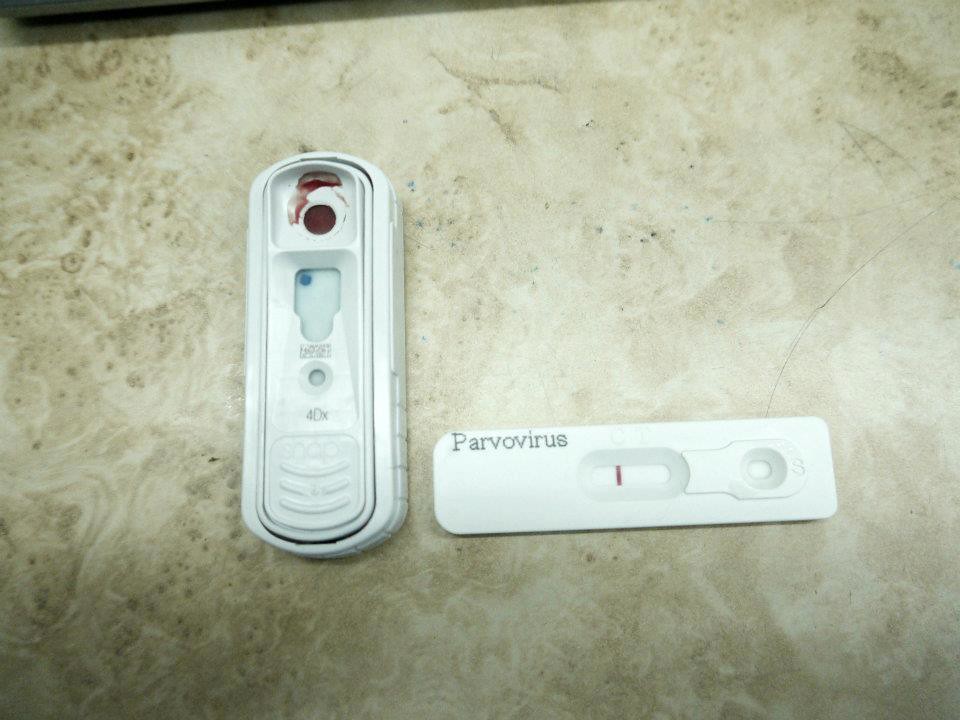The image showcases two medical test devices made of plastic. Both devices feature a tan surface with intricate, darker tan patterns. 

The first device is positioned vertically and has a long, oval shape. It contains an oval within an oval, with a rectangle at its center. Above this rectangle, there is a dark red spot, potentially indicative of blood. Additionally, there is a dark red circle accompanied by a corresponding dark red smear on the plastic. On the other side of the oval, three small, upraised lines draw attention. In the middle section, a small circle is observed alongside a small square, which together form a diminutive screen displaying a minor blue dot.

The second device, lying horizontally beside the first, is also long and oval but smaller in size. This test is labeled "Parvovirus". It features an oval central section marked by a single red line. Adjacent to this is a small circle situated above another smaller circle, emblazoned with a letter "S". To the right of the red line, the letters "C" and "T" are inscribed vertically.